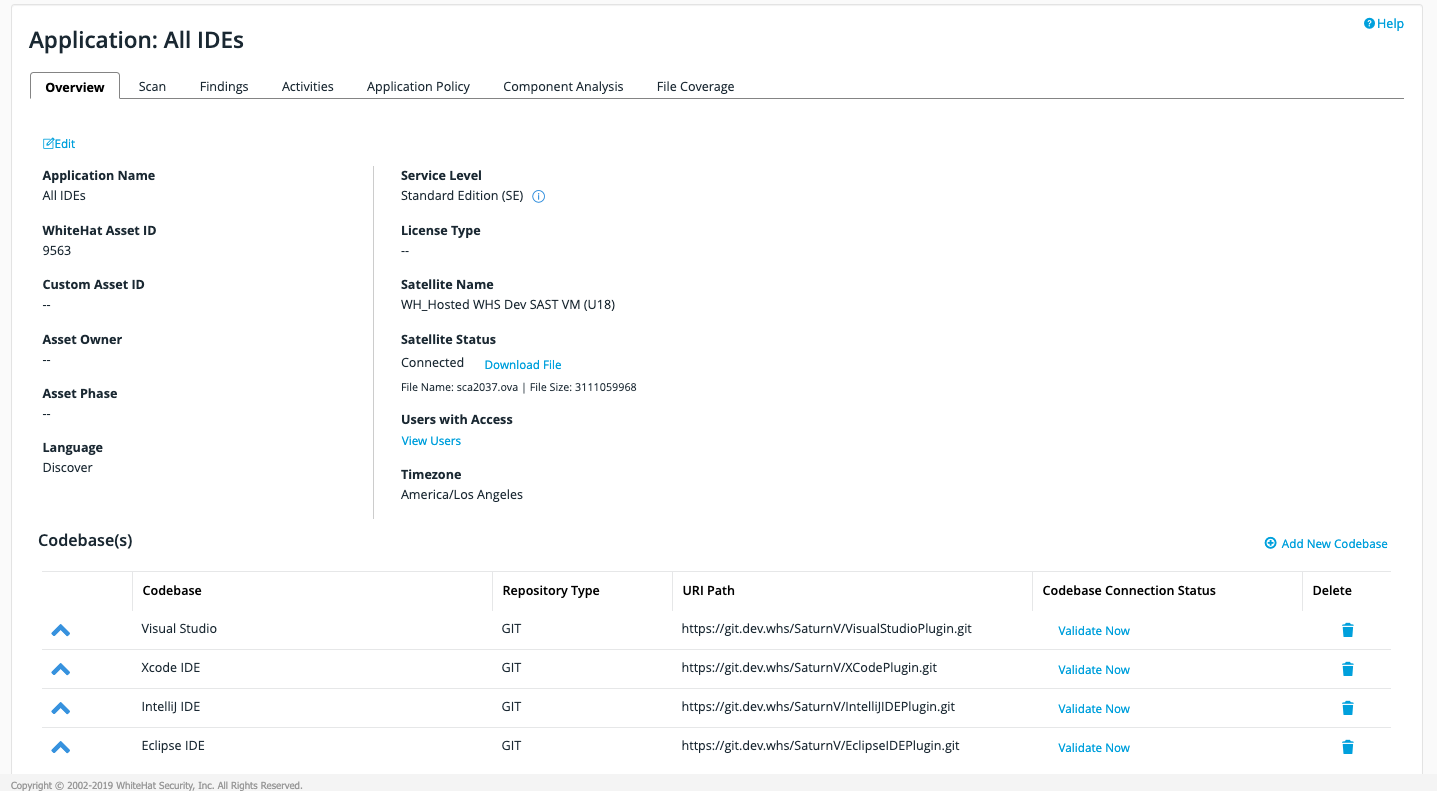This image contains an interface screenshot filled with extensive information and several interactive elements. At the top left, written in black text, is the label "Application (all IDEs)" where 'IDEs' is uppercase, and the 's' is lowercase. Below this label are various tabs to choose from: Overview, Scan, Findings, Activities, Application Policy, Component Analysis, and File Coverage. The "Overview" tab is highlighted, indicating it is currently selected.

Below the tabs, there are two lists of detailed information. On the left side of the interface, "Application Name" is displayed, and on the right side, "Service Level" is indicated. Further down, a section titled "Code Bases" is displayed, with the 's' at the end in parentheses (indicating potential plurality). To the right of this section title, there is a clickable blue link prompting the user to "Add a New Code Base."

Underneath this header, there is a list featuring four distinct code base entries. For each entry, several columns of information are provided: Code Base, Repository Type (spelled out as "R-E-P-O-S-I-T-O-R-Y"), URI Path, Code Base Connection Status, and an option to delete the code base entry.